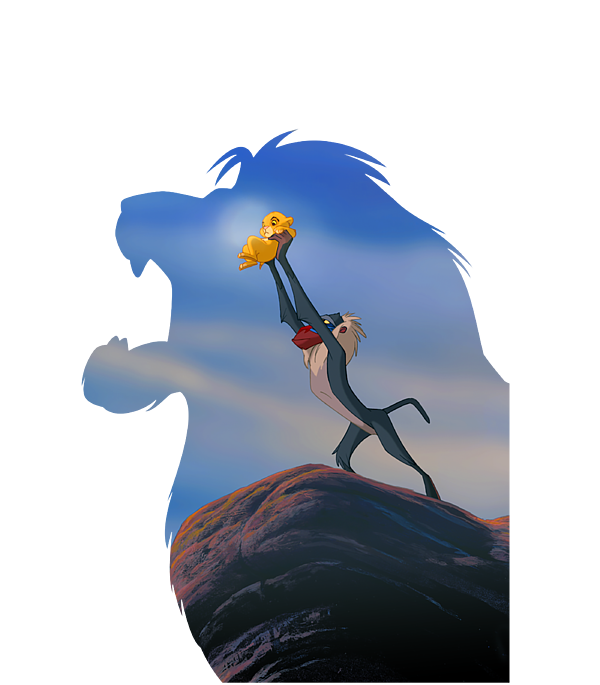This image is a detailed artistic rendition inspired by Disney's The Lion King. It features Rafiki, the eccentric baboon with a distinctive white beard and bright red and blue facial markings, ceremoniously holding up the young lion cub, Simba, atop the iconic Pride Rock. This pivotal moment, integral to the movie, is creatively overlaid onto a larger silhouette of an adult Simba, depicted in a roaring pose. The silhouette is rendered in shades of sky blue, encapsulating the scene within its contours. The background is filled with vibrant colors of the sky and clouds, adding depth to the composition. The lower part of the image showcases the majestic rock outcropping in hues of orange, green, and pink, gradually darkening as it descends, grounding the legendary moment in the grandeur of the African savannah.